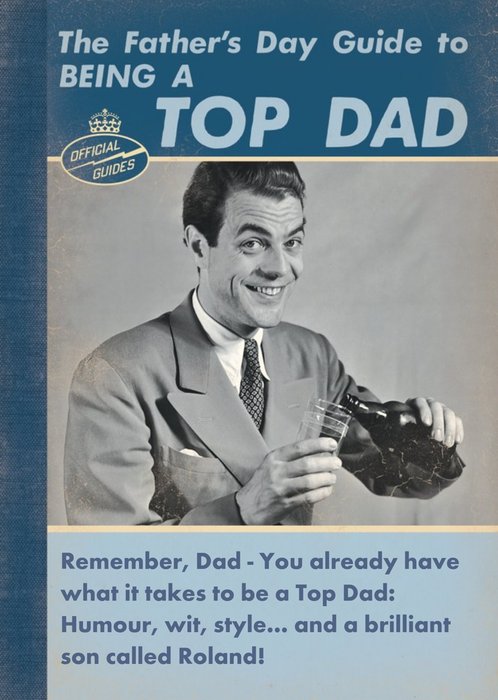This image resembles the cover of a vintage magazine or book titled "The Father's Day Guide to Being a Top Dad." The background features a combination of dark and light blue hues. At the top, in large light blue letters against a dark blue backdrop, the title is prominently displayed. Just below, there is a small crown symbol accompanying the words "Official Guides."

The centerpiece of the cover is a black and white photograph of a smiling, clean-shaven, middle-aged man with short black hair. He exudes happiness as he looks directly at the camera. The man is elegantly dressed in a suit, complete with a shirt, tie, and a pocket square. He is depicted pouring a drink from a bottle, held in his left hand, into a glass cup in his right hand.

Below the photograph, in dark blue text against a light blue background, the caption reads: "Remember, Dad, you already have what it takes to be a top dad. Humor, wit, style, and a brilliant son called Roland." This detailed composition emphasizes both the stylish appearance of the man and the heartfelt message about fatherhood.